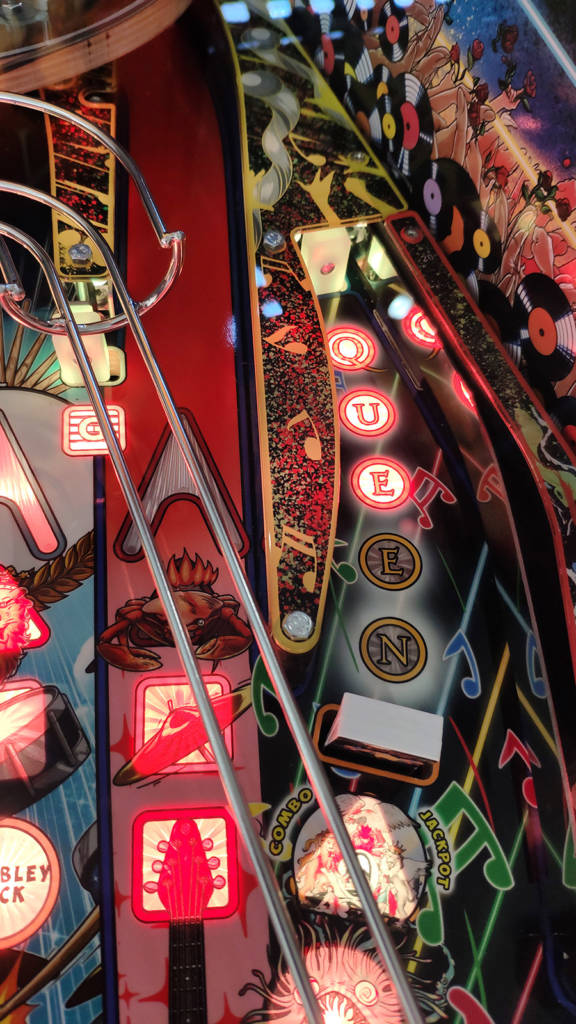This detailed and vibrant photograph captures a zoomed-in section of a Queen-themed pinball machine. Dominating the background are striking, colorful elements with vivid lights and intricate designs, emphasized by the bright and varied artwork. Central to the composition are individual circles spelling out "Q-U-E-E-N," with the letters Q, U, and E illuminated, and the letters arranged vertically with a slight curve. Surrounding the letters are musical motifs, including red, blue, and green notes, as well as a picture of the top of an electric guitar with red detailing and a black strip at the bottom, adding to the rock 'n' roll aesthetic.

Further enhancing the intricate visual appeal, the machine features a crab seemingly on fire perched atop a red square frame, iconic symbols like drum kit elements and a hi-hat, and other thematic images such as a grain of wheat and a sun. The metallic silver railing for the ball curves from the bottom up and to the left, merging into a chute—signifying the pathway for the actual gameplay.

In the background, captivating imagery depicts vinyl records and a crowd of people at a concert, reinforcing the music and band theme. Text elements like "COMBO" and "JACKPOT" add to the gaming context of the pinball machine. The detailed artwork, combined with the bright lights and reflective accents, culminates in a visually rich snapshot of this tribute to the legendary band Queen.